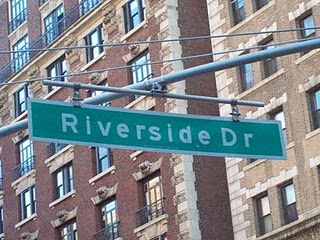This daytime photograph captures a green street sign with white lettering that reads "Riverside Drive," mounted on a sleek silver metal pole. In the background, two closely situated brick buildings dominate the scene. One building boasts a rich, orange-hued brick facade, while the other showcases a mid-tone tan brick exterior. Multiple windows adorn both structures, some of which have bars over them, while the sunlight glistens off several other window panes. The image quality is exceptionally clear and crisp, allowing for easy discernment of intricate details.